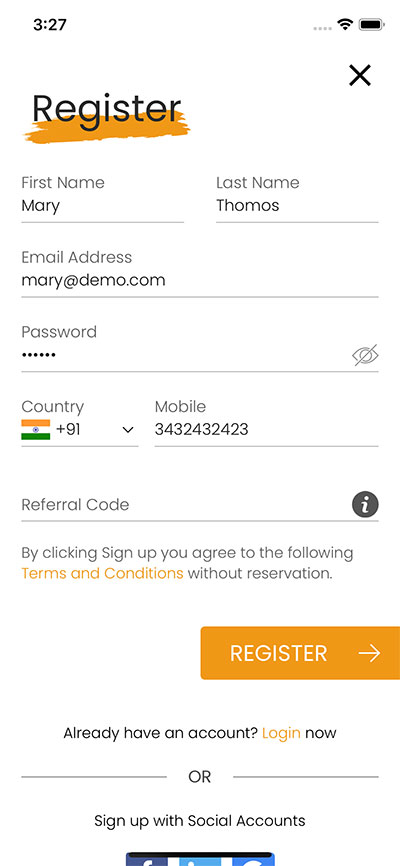The image appears to be a screenshot of a registration page on a mobile device, evident from the typical mobile UI elements at the top, such as the battery icon, Wi-Fi signal indicator, and the time displayed as 3:27 in the upper left corner. The page is predominantly white, featuring black text and accented with orange elements.

At the top of the screen, there's a header with the word "Register" prominently displayed in black text, accompanied by an orange marker. Below the header, there are various input fields for user information:

1. **First Name:** Mary
2. **Last Name:** Tomas
3. **Email Address:** mary@demo.com
4. **Password:** [hidden in the image]
5. **Country:** Indicated by an orange, white, and green flag, probably representing India. The country code is +91.
6. **Mobile Number:** 343-243-2432
7. **Referral Code:** Optional, with an information icon for help.

At the bottom of the form, there is a disclaimer stating, "By clicking Sign Up, you agree to the following terms and conditions without reservation." This is followed by an orange "Sign Up" button with white text.

Further down, there's a prompt that says, "Already have an account? Log in now," and an option to "Sign up with social accounts," though some social account options are partially cut off in the image. The screenshot gives a comprehensive view of the registration section, detailing the various fields for input and highlighting the main actions users can take.